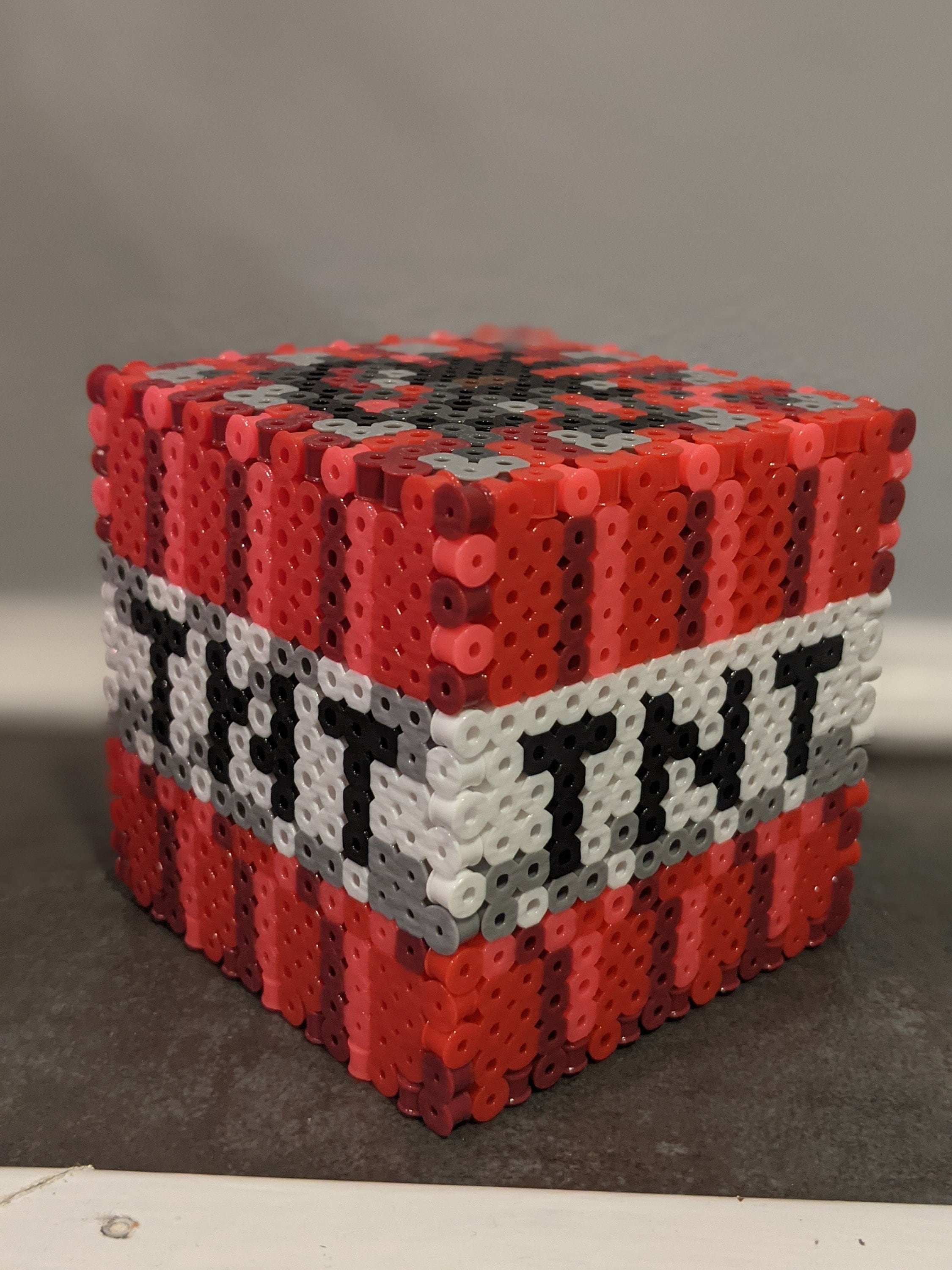The image features a block constructed to resemble TNT dynamite. It appears to be made up of tiny, cylindrical pieces, akin to pencil erasers, which seem to be solid plastic. These small pieces come in varying shades of red—from dark to medium and light red—and they meticulously form the overall shape of the block. A distinctive band wraps around the center, crafted from white and gray pieces, bearing black letters that spell out "TNT" on two of its sides. The block sits on a black flat surface, and the image, characterized by a high depth of field, reveals a blurred gray foreground and a white border in the background, enhancing the impression of an abstract, pixelated composition.